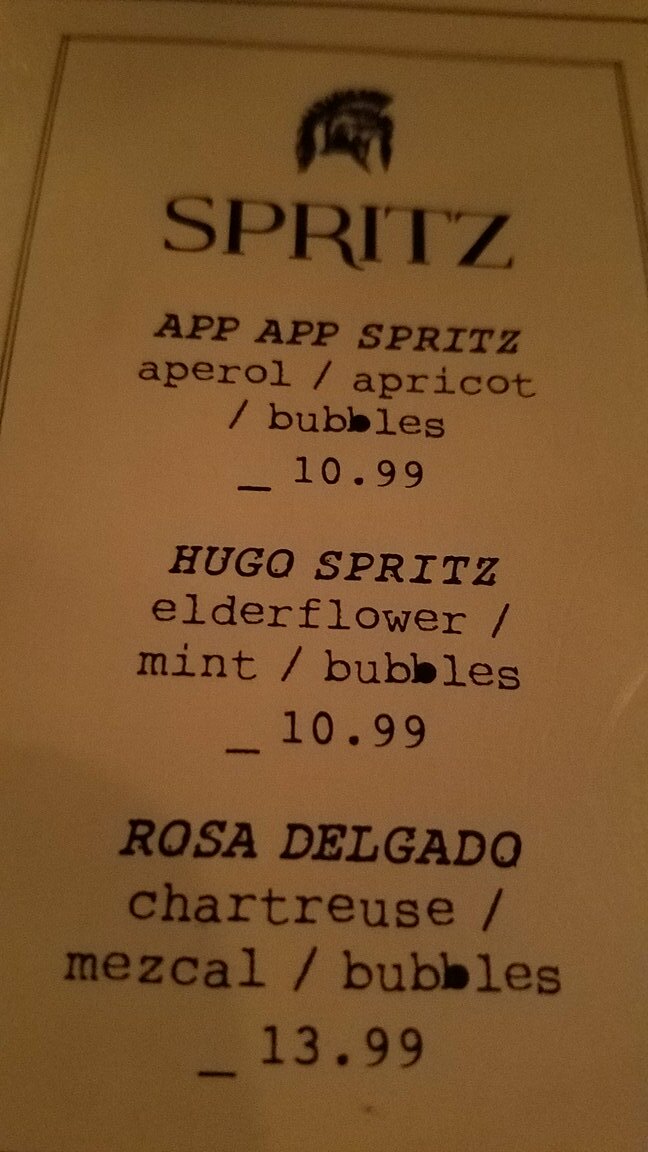This is a high-resolution photograph of a simplistic yet elegant menu. The menu itself is a long, white piece of cardstock with a subtle glossy finish that gives it a slightly reflective quality. It is bordered on the right side by a thin band of gold, adding a touch of sophistication to the minimalist design.

Prominently displayed at the top in large, bold, black capital letters is the word "SPRITZ". Directly below this heading is an intricately designed emblem that resembles a helmet with a prominent mohawk, suggestive of strong, perhaps Roman or gladiatorial, imagery.

The menu lists a selection of drinks, each detailed with ingredients and prices. It features:

- **Aperol Spritz**: described as Aperol, apricot, and bubbles, priced at $10.99.
- **Hugo Spritz**: a combination of elderflower, mint, and bubbles, also $10.99.
- **Rose Delgado**: a more elaborate mix of Chartreuse, Mezcal, and bubbles, priced at $13.99.

The photo captures the menu with some visible shadows cast across it, indicating that the image was taken in a dimly lit, possibly intimate setting. The overall image quality is somewhat grainy, suggesting a low-light environment which adds a sense of ambiance to the scene.